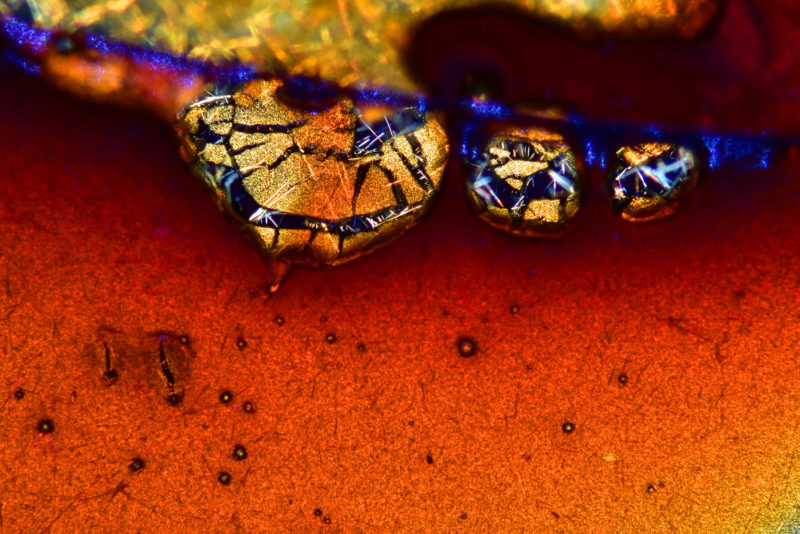This highly magnified image seems to showcase an abstract and detailed close-up, making it difficult to pinpoint the subject exactly. The lower half of the image reveals a textured surface with an orange-hued material, speckled with black dots, resembling discolored skin or perhaps an insect wing. At the bottom right, a small yellow and green marking stands out against the intricate background. Moving upwards, the central portion features three distinct, jewel-like droplets that appear gold with blue cracklings and sparkling black cracks running through them. These "jewels" vary in size, with the largest on the middle left, a medium-sized one to its right, and the smallest further right. The upper section of the image transitions into a blurred background with a golden, thread-like appearance and a distinctive blue sparkly line cutting across diagonally from the top left. Overall, the image combines elements of organic textures and what seems to be ornamental details, all through a lens of high magnification.